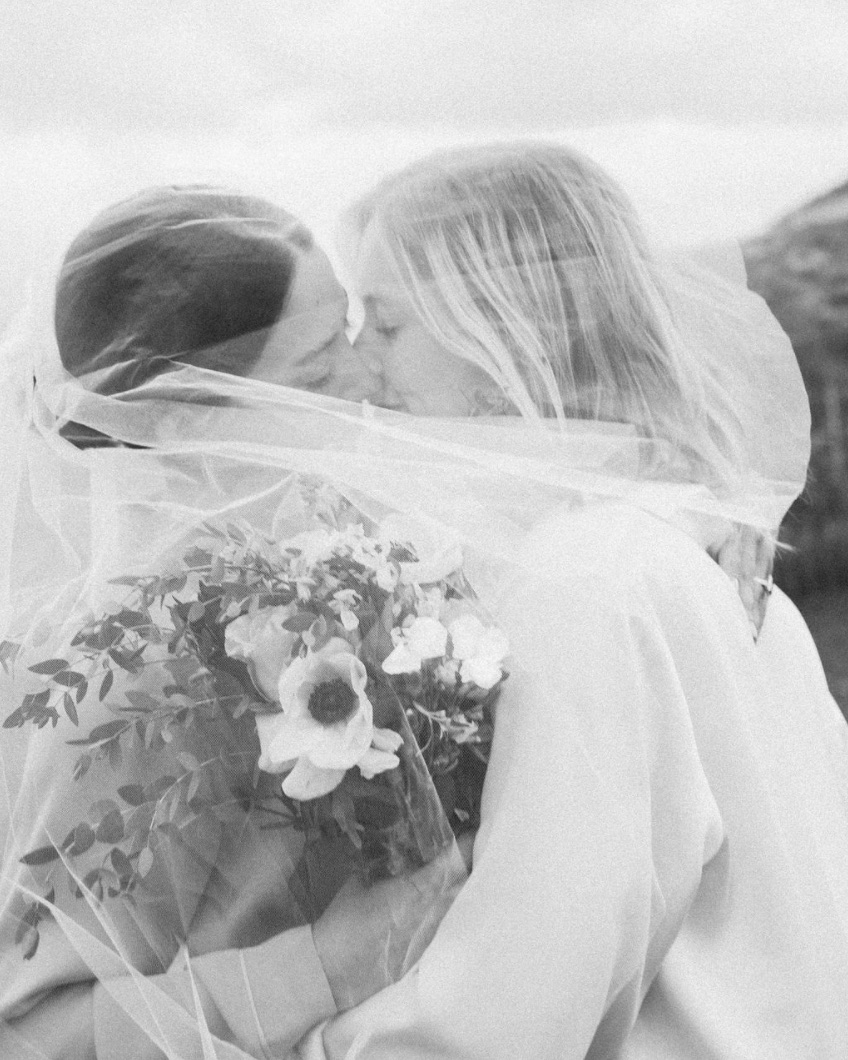This black-and-white photograph depicts a tender moment between two women, seemingly captured on their wedding day. They share a kiss under a delicate, translucent gauze veil, reminiscent of tulle. The woman on the left, with her dark hair elegantly pulled back, cradles a bouquet of large flowers, possibly carnations and leaves. She tenderly wraps her arm around her partner's shoulder. The woman on the right, with shoulder-length hair featuring blonde tips, embraces her partner by the waist. Both are dressed in light, long-sleeved attire, contributing to the ethereal quality of the scene. The blurred background suggests a gray sky with clouds, adding to the timeless romantic atmosphere of the image.